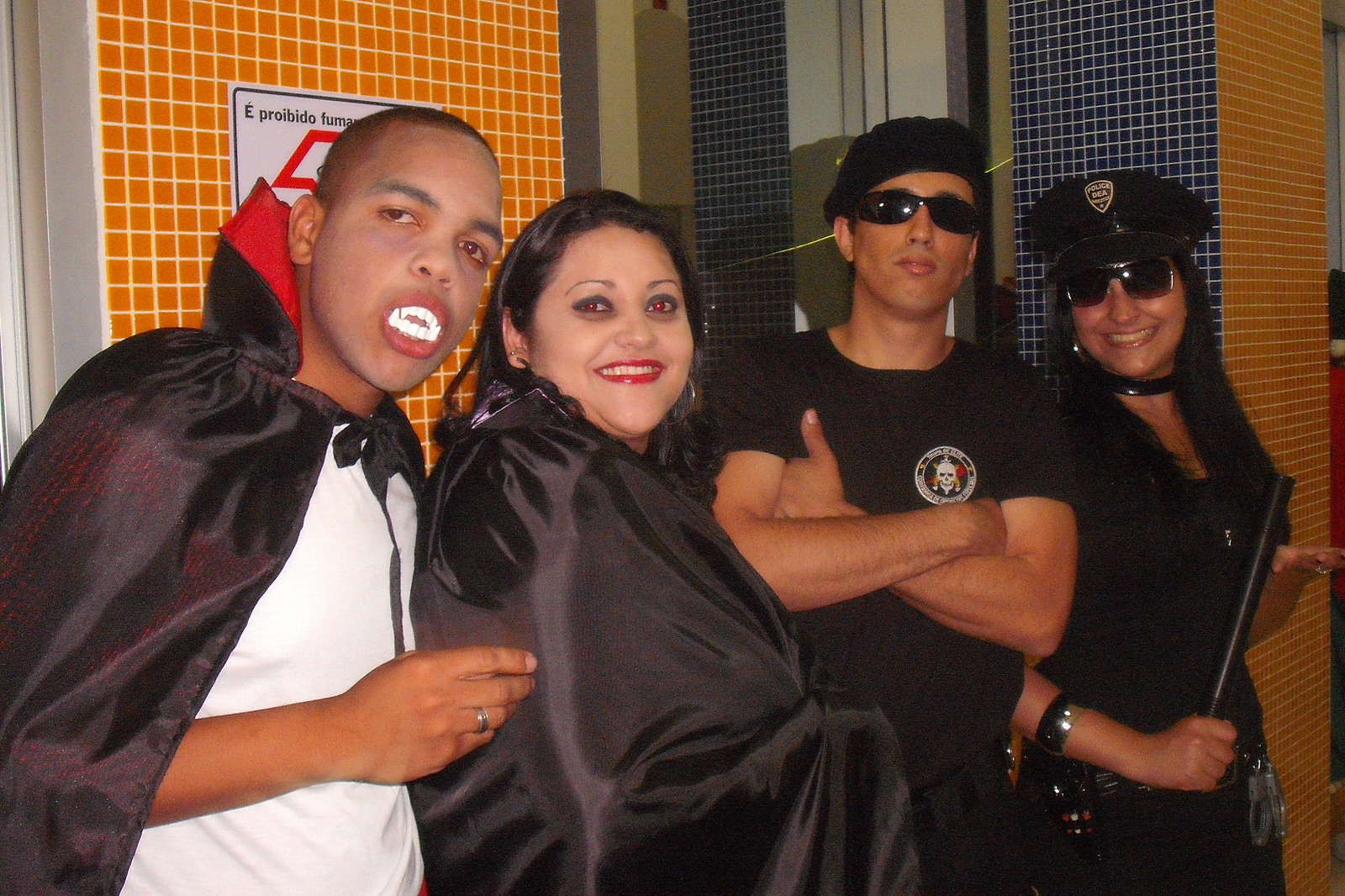This detailed photo captures four young individuals, seemingly in Halloween costumes, standing side by side in front of a tiled wall adorned with orange and blue tiles, partially obscured by a sign reading "Iproibido" and "Fuma." On the far left, a man dressed as a vampire sports fake fangs, a dramatic Dracula cape, and a white shirt, while leaning towards the woman next to him. She appears with heavy dark eye makeup, bright red lips, and dark hair, wrapped in a black cloak, possibly hinting at a vampire theme as well. To her right stands a man in a black t-shirt featuring a skull badge, arms crossed and hands tucked in, complemented by a black beret and black sunglasses. The woman beside him is dressed as a police officer with a matching cap and is holding a nightstick, smiling brightly for the camera. It seems they all are posing against the backdrop of a tiled wall with columns, creating an engaging and festive Halloween scene.